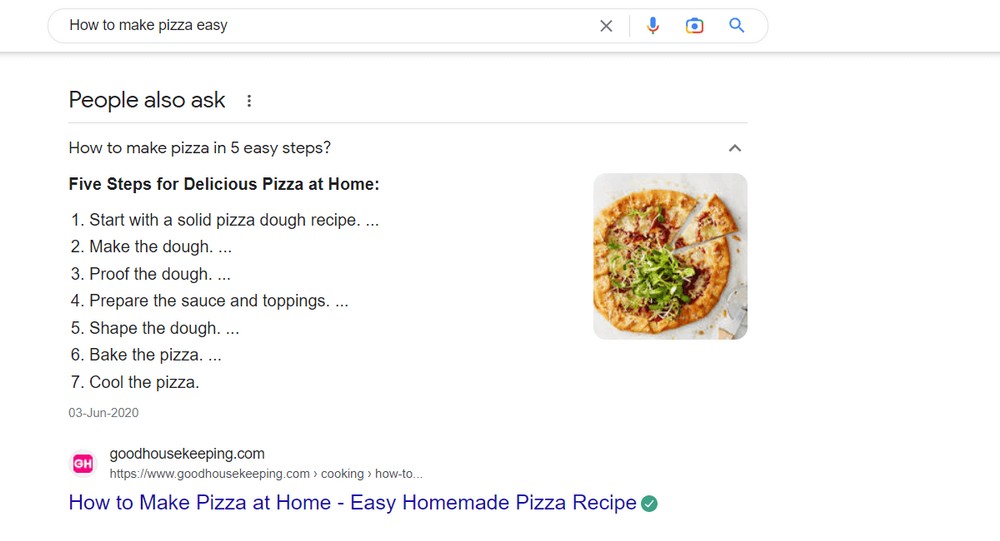On a crisp white background, the search interface is displayed prominently. At the top, there’s a search bar where the phrase "how to make pizza easy" is typed in black text. To the right of the search bar, icons are aligned, including a gray "X" (to clear the search), a colorful microphone (for voice search), a small blue camera icon (to search with an image), and a blue magnifying glass icon (to execute the search).

Below the search bar is a gray dividing line. Underneath this line, there are search suggestions listed under the heading "People also ask," written in black text. The first suggestion reads "How to make pizza in five easy steps," followed by detailed instructions:

1. Start with a salad pizza dough recipe.
2. Make the dough.
3. Proof the dough.
4. Prepare the sauce and toppings.
5. Shape the dough.
6. Make the pizza.
7. Cool the pizza.

Beneath these steps, in gray text, the date "03 Jun 2020" is noted, followed by the source listed twice: "goodhousekeeping.com." Directly next to this, in blue, a clickable link states: "How to make pizza at home – Easy homemade pizza recipe," accompanied by a teal circle with a white check mark.

On the far right-hand side of the layout, a visually appealing pizza is showcased. The pizza has a beautifully golden crust and is generously loaded with various toppings. However, only one slice has been taken out, and it appears the slice was not fully cut, as none of the toppings in the center are disturbed—clearly arranged for an ideal photo opportunity.